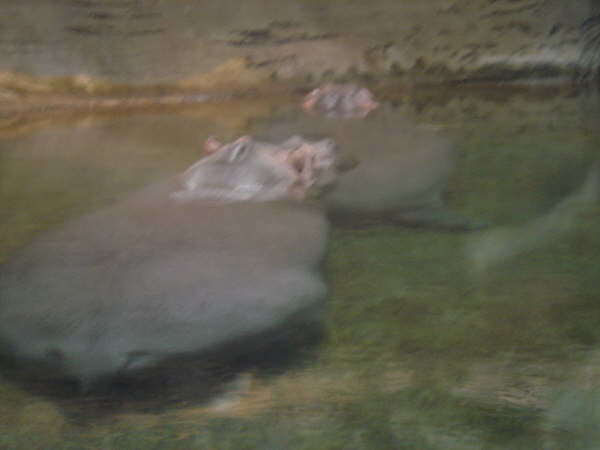The image shows a blurry view of what appears to be an animal enclosure with water at the bottom. The enclosure, primarily brown in color with some artificial-looking stones or platforms, features the presence of two indistinct creatures that are difficult to identify due to the blurriness and poor focus. The creatures could possibly be hippopotamuses; one seems to have a lighter-colored head with small ears and a snout pointing towards the upper right. There’s another similar creature further in the distance, and its features are obscured. Amidst the scene, there are patches of gray and khaki green, which might indicate additional elements in the enclosure or distant fields, with a hint of yellow possibly marking the edge of the area. The overall lack of clarity makes it challenging to discern specific details of the setting or the animals.